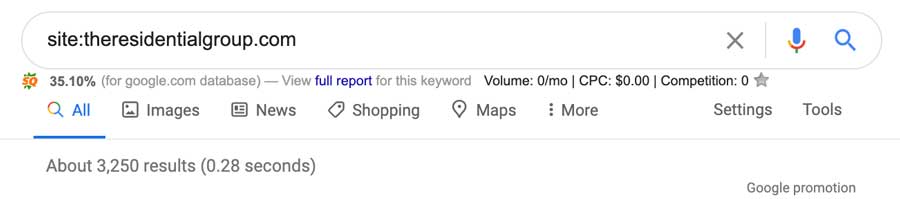This is a cropped screenshot of a Google search results page. The top, left side, and bottom of the website are cropped out, but the search bar is still visible at the top. Inside the search bar, the query "site:theresidentialgroup.com" is entered. Below the search bar on the left, there's a small yellow icon displaying the number "50." To the right of this icon, "35.10%" is shown in gray, followed by text in parentheses that reads "for google.com database."

Adjacent to this, the text "View full report for this keyword" appears, with "Full report" hyperlinked. Moving further to the right, it states "Volume $0 a month, CPC," followed by a dollar sign and "$0." Next, there's information on "Competition," marked as "zero," accompanied by a small, grayed-out star icon.

Below this section, a list of categories is displayed horizontally: "All," "Images," "News," "Shopping," "Maps," "More," "Settings," and "Tools." Underneath these categories, the search results indicate about "3,250 results" in "0.28 seconds." At the very bottom right of the screenshot, in very small gray letters, is the text "Google promotion."